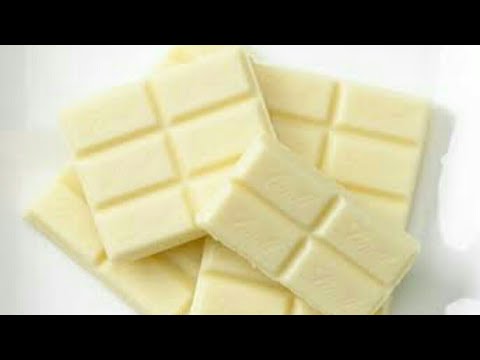This image depicts a stack of rectangular pieces of white chocolate arranged haphazardly on a white surface with wide, black rectangular bars at both the top and bottom of the frame. The top piece of chocolate, consisting of 2x2 squares, is oriented southeast. Below it is a 2x3 piece, and beneath that is a larger piece similar in size to the one underneath it, which has 4x3 squares; the exact number of segments on the bottom piece is not visible but appears comparable in size. Throughout the stack, each piece is divided into smaller rectangular blocks. There is faint, potentially illegible text on the chocolate pieces and some squiggly lines, though it's unclear if these are part of the chocolate design or a visual aberration. A slight, light gray shadow is cast on the right side of the stack, adding a subtle depth to the composition.